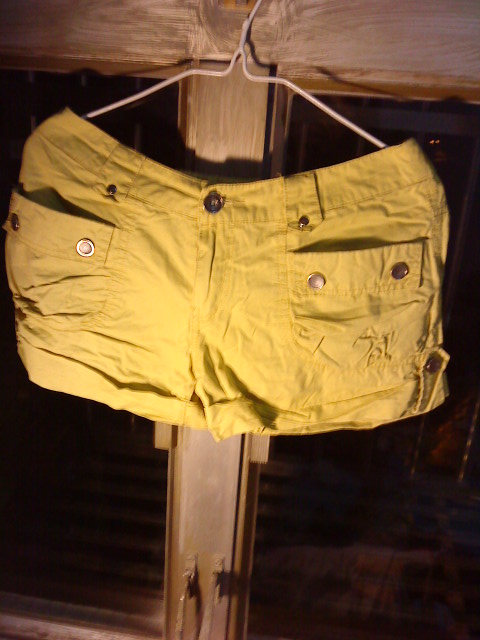The image depicts a pair of mustard yellow jean shorts hanging on a white metal wire hanger, which is hooked over the waistband. The shorts are the focal point, positioned top-center of the portrait-oriented photograph. The backdrop appears to be a dark window frame with wooden vertical and horizontal elements, suggesting the shot was taken at night or in a dimly lit room. The shorts feature a button and zipper closure at the waist, along with two front pockets each adorned with pearlescent, metal reflective studs. These pockets include a small design, especially noticeable on the right pocket. The shorts also have belt loops and a cuffed hem, with visible creases indicating they have been worn or are not freshly ironed. The camera's flash seems to have been used, as evidenced by the subtle highlights on the left bottom quarter of the shorts, which enhances their mustard hue and the reflective details. The hanger is sturdy, supporting the lightweight, possibly cotton fabric of the shorts. The window frame has two handles at the bottom, pointing outward, adding to the depth and context of the scene.